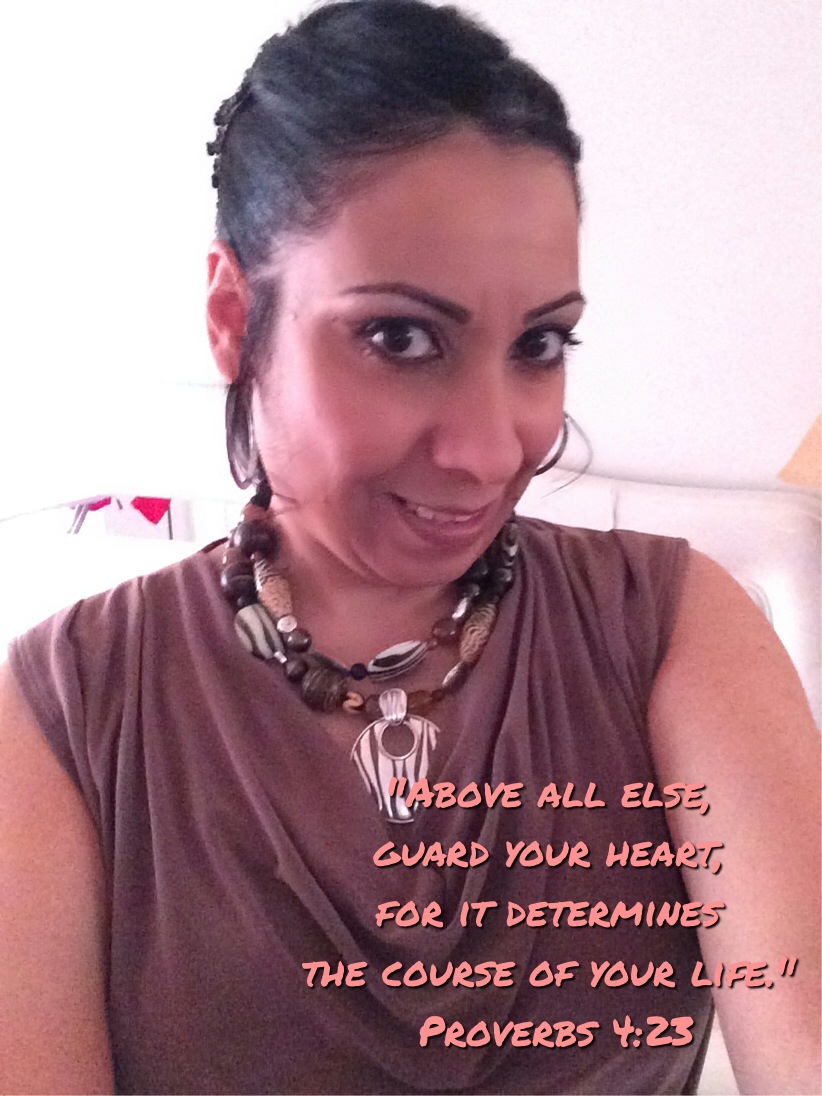This image captures a woman, who appears to be in her thirties, with dark hair pulled back from her face, emphasizing her dark eyes and lightly made-up features, including orange-tinted eyebrows. She has a slight smile, with her chin gently resting against her neck. She is wearing a sleeveless brown dress with a cowl neck, and a prominent beaded necklace featuring a large pendant. The photograph is a selfie, cut off just below her chest, and shows both her arms at her sides. In the bottom right corner of the image, there is an inspirational quote from Proverbs 4:23, displayed in orange, all-capital letters: "Above all else, guard your heart, for it determines the course of your life." She is posed indoors, with a white sofa visible in the background.